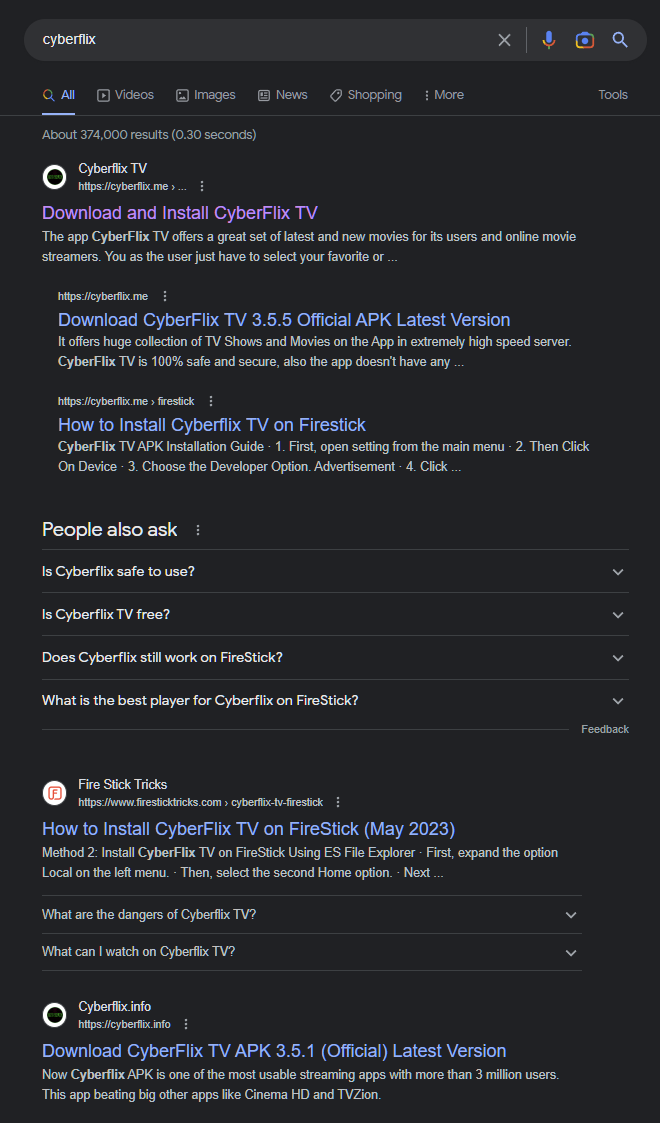### Detailed Caption:
The image captures a Google search result page for the query "Cyberflix," spelled C-Y-B-E-R-F-L-I-X. Within 0.3 seconds, approximately 374,000 results were generated. The top search result is titled "Cyberflix TV," accompanied by a succinct subtitle encouraging users to "Download and install Cyberflix TV." The meta description reads: "The app Cyberflix TV offers a great set of latest and new movies for its users and online movie streamers. You as the user just have to select your favorite..." but it truncates there. Nested under the main link are two additional links: "Download Cyberflix TV 3.5.5 Official APK Latest Version" and "How to Install Cyberflix TV on Firestick." 

Further down, the "People also ask" section is visible, featuring four expandable questions:
1. Is Cyberflix safe to use?
2. Is Cyberflix TV free?
3. Does Cyberflix still work on Firestick?
4. What is the best player for Cyberflix on Firestick?